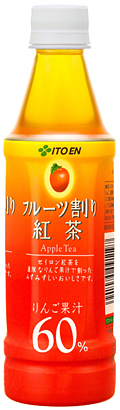The image features a small beverage bottle with a variegated color scheme, transitioning from yellow at the top to red at the bottom. The bottle has a white twist-off cap. The label includes black lettering spelling out "ITO EN" to the right of four green circles arranged in a square. Predominantly, the label has a light orange hue with white text featuring the term "apple tea" amid Chinese or Japanese writing. Prominently displayed on the bottom portion of the label is "60%" in white on a red background. A partially visible UPC code and a small green bar are located at the bottle’s base. The label also depicts a red fruit, likely a tomato, with green leaves on top.